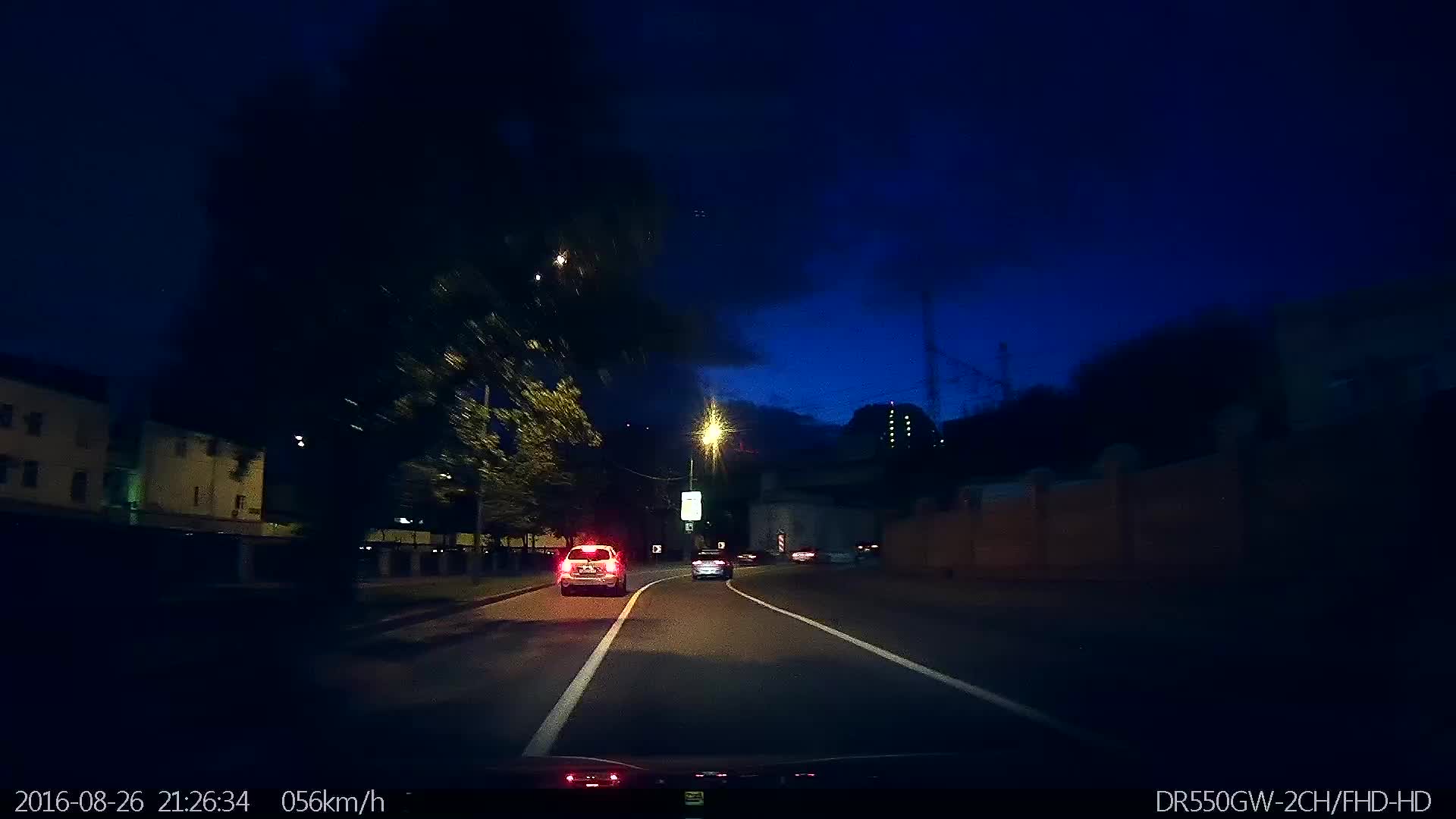A captivating night-time dash cam capture reveals a moody, purplish-blue sky adorned with faint, wispy clouds. The road stretches ahead, marked by two distinct lines separating the lanes. In the foreground, multiple cars are visible, their red taillights forming a vivid contrast against the dark surroundings. A solitary vehicle cruises in the opposite lane, adding to the dynamic movement of the scene. Illuminated by a prominent streetlight at the center, the image also features smaller, ambient lights near a partially-lit tree to the left. To the right, a building stands dimly lit, adding an urban touch to this nocturnal snapshot.